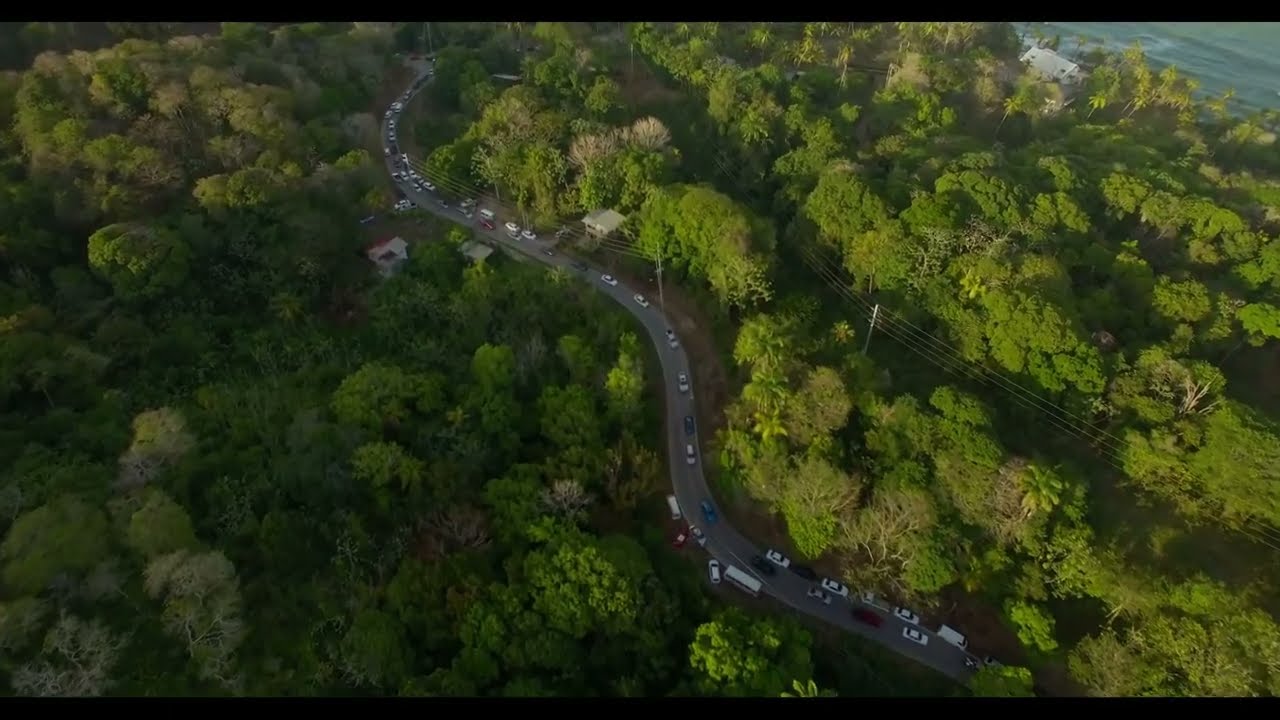This overhead photograph, likely taken by a drone or an airplane, showcases a densely forested area, possibly a park or a forest, blanketing the entire image with lush green canopies. The view is strictly downward with no sky in sight, emphasizing the expansive cover of trees that stretch from edge to edge. Notably, the lower left section of the forest is cast in shadow, while the upper right to right center areas are bathed in sunlight.

Bisecting this verdant landscape is a winding, four-lane paved asphalt highway that snakes its way diagonally from the upper left center to the lower right of the image. The road appears to be heavily trafficked, particularly on the right side lanes. Scattered among the trees are a few small cottages, houses, and visible power lines, yet these structures are minimal compared to the overwhelming presence of the forest.

Adding a final touch to the composition, the very tip of the upper right corner reveals a small portion of a blue water body, likely a lake or the sea, accompanied by what appears to be a beachfront home. The photograph captures the contrast between the tranquility of nature and the bustling activity on the highway below, all under the bright daylight.